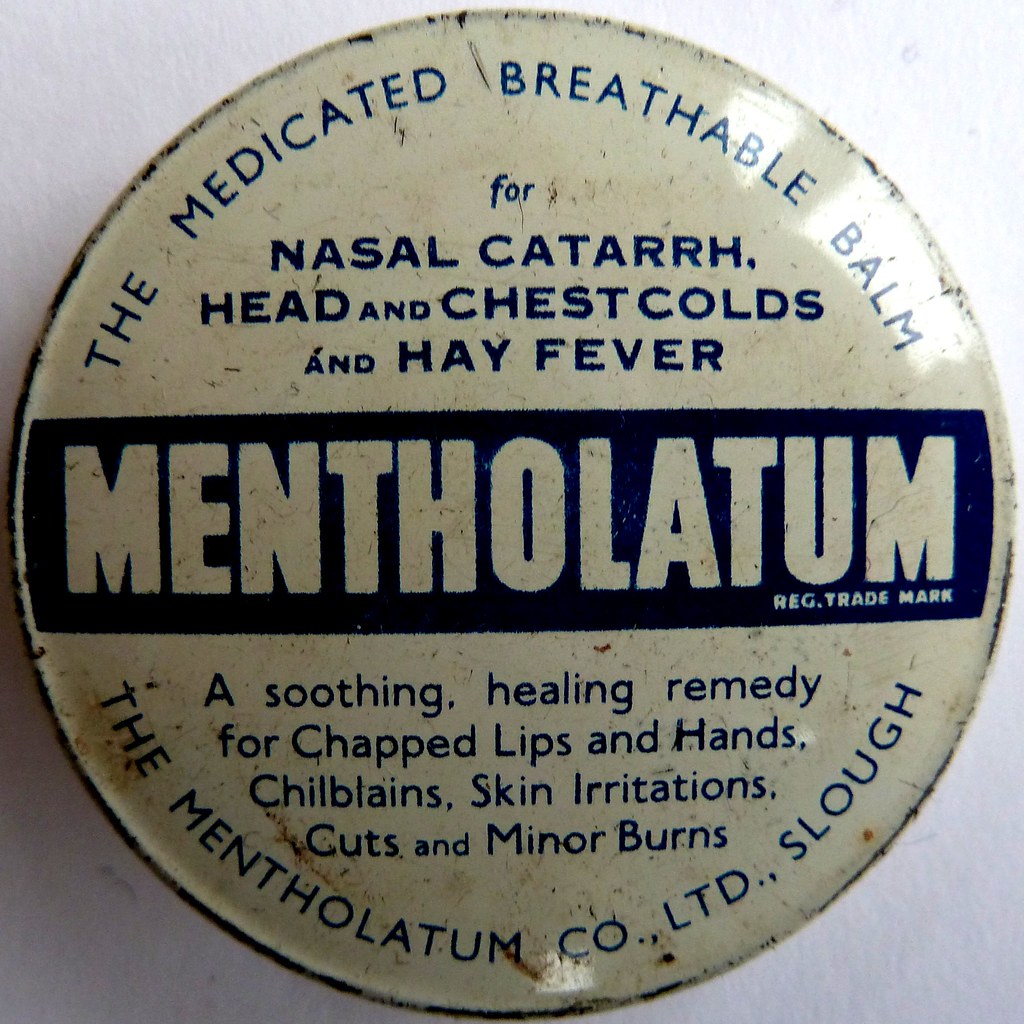This image features a close-up of an old, round, and worn metal tin of Mentholatum rub placed on a white table. The tin, which is off-white with a dark blue rectangular centerpiece, shows signs of age with multiple scratches, dings, and spots of rust. The top of the tin prominently displays "Mentholatum" in white block letters within the blue rectangle, accompanied by "REG. trademark" beneath it. Encircling the top edge, the text reads "The medicated breathable balm for nasal catarrh, head and chest colds, and hay fever," while along the bottom edge it states "A soothing, healing remedy for chapped lips and hands, chilblains, skin irritations, cuts, and minor burns." Additionally, at the very bottom, it notes "The Mentholatum Company Limited, Slough." This well-used tin reflects its longevity and the trust placed in its contents over the years.